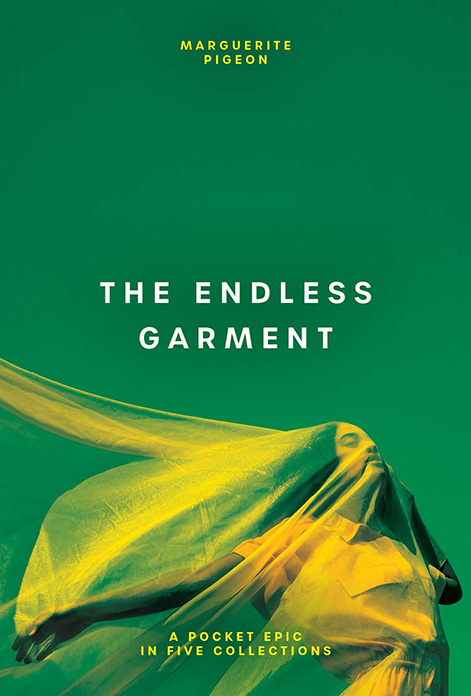This book cover features a solid medium-dark green background. At the top, the author's name, "MARGUERITE PIGEON," is prominently displayed in bold, capital yellow letters. Centered in the middle of the cover, the title "THE ENDLESS GARMENT" appears in bold, white capital letters with the words slightly spaced apart for emphasis. 

Beneath the title, an image captures a girl facing left, enveloped in a transparent garment that is billowing in the wind. The sheer veil covers her entire body and head, flowing behind her to the right, with one of her arms partially caught in the fabric. She appears to be wearing a yellow outfit underneath the veil. 

Towards the bottom middle of the cover, the words "A POCKET EPIC IN FIVE COLLECTIONS" are inscribed in capital yellow letters, completing the design. The overall layout indicates this is the front cover of a book, emphasizing a harmonious blend of green, yellow, and white hues.